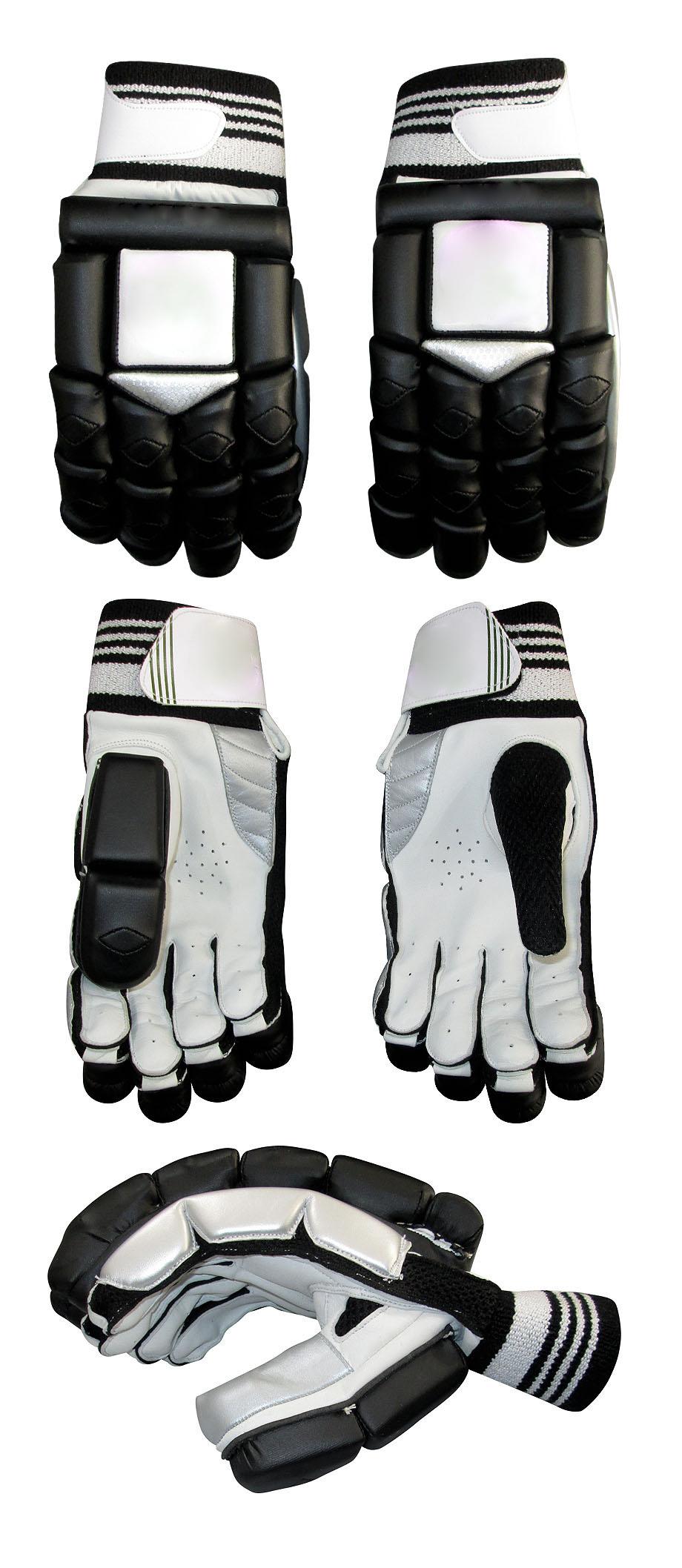This image features three pairs of sports gloves neatly arranged against a white background. The topmost pair displays a striking combination of black and white leather-like material. The gloves' wrist cuffs are white with black stripes, leading to a black hand area adorned with white decorative elements and diamond shapes on the knuckles. The middle pair is predominantly white, crafted from a leather-like fabric, with a black thumb featuring a diamond decoration. Their wrists match the top pair with white and black striped cuffs, black fingertips, and a white back. Below these pairs is a single, heavily padded glove. This glove is primarily black with white and black padding over the fingers and the back of the hand. Its wristband is made of white fabric, also featuring black and white stripes. The gloves are displayed from different angles, including palm down, palm up, and a side view, highlighting the thick, blocky cushioning. These gloves appear highly protective, likely designed for a high-contact sport such as hockey. They include features like breathable holes and Velcro straps for secure fitting.